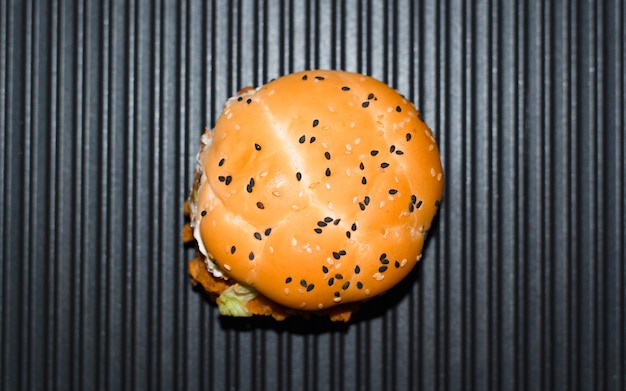This detailed photograph features a round, light brown hamburger bun with distinctive folding lines and a mix of black and white sesame seeds generously sprinkled across its surface. The bun sits atop a dark grey, metallic surface characterized by vertical grooves, resembling a grill top. In the bottom left corner, a piece of green lettuce peeks out, along with what appears to be a piece of crispy chicken slightly dangling from the side. A hint of white, likely mayonnaise or onion, is also visible on the side. The rectangular image is captured in landscape orientation, with the bun prominently centered amidst the dark, grooved background.